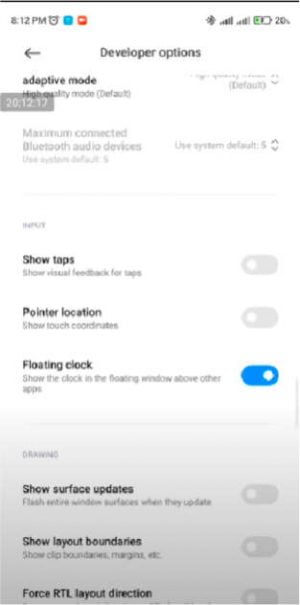Screenshot of the Developer Options Page:

Displayed in a light gray to white gradient background, this screenshot features the "Developer Options" page of a settings interface. At the very top, there's a navigation bar with a left-pointing back arrow. Centrally positioned is the heading "Developer Options" in bold text. 

Briefly beneath this heading, the first option listed is "Adaptive Mode" with a description indicating it is "High Quality Mode (Default)". Below this is the "Maximum Connected Bluetooth Audio Devices" option. Separating these sections is a horizontal line divider.

The next section, labeled "Inputs," includes three toggle options:
1. Show Tips - toggled off (gray)
2. Point to Location - toggled off (gray)
3. Floating Clock - toggled on (blue)

Another section follows, but its title is too blurry to read. Here, three more toggle options are listed:
1. Show Surface Updates - toggled off (gray)
2. Show Layout Boundaries - toggled off (gray)
3. RTL Layout Direction - toggled off (gray)

The detailed layout and color indicators allow users to easily identify and navigate through various developer settings.